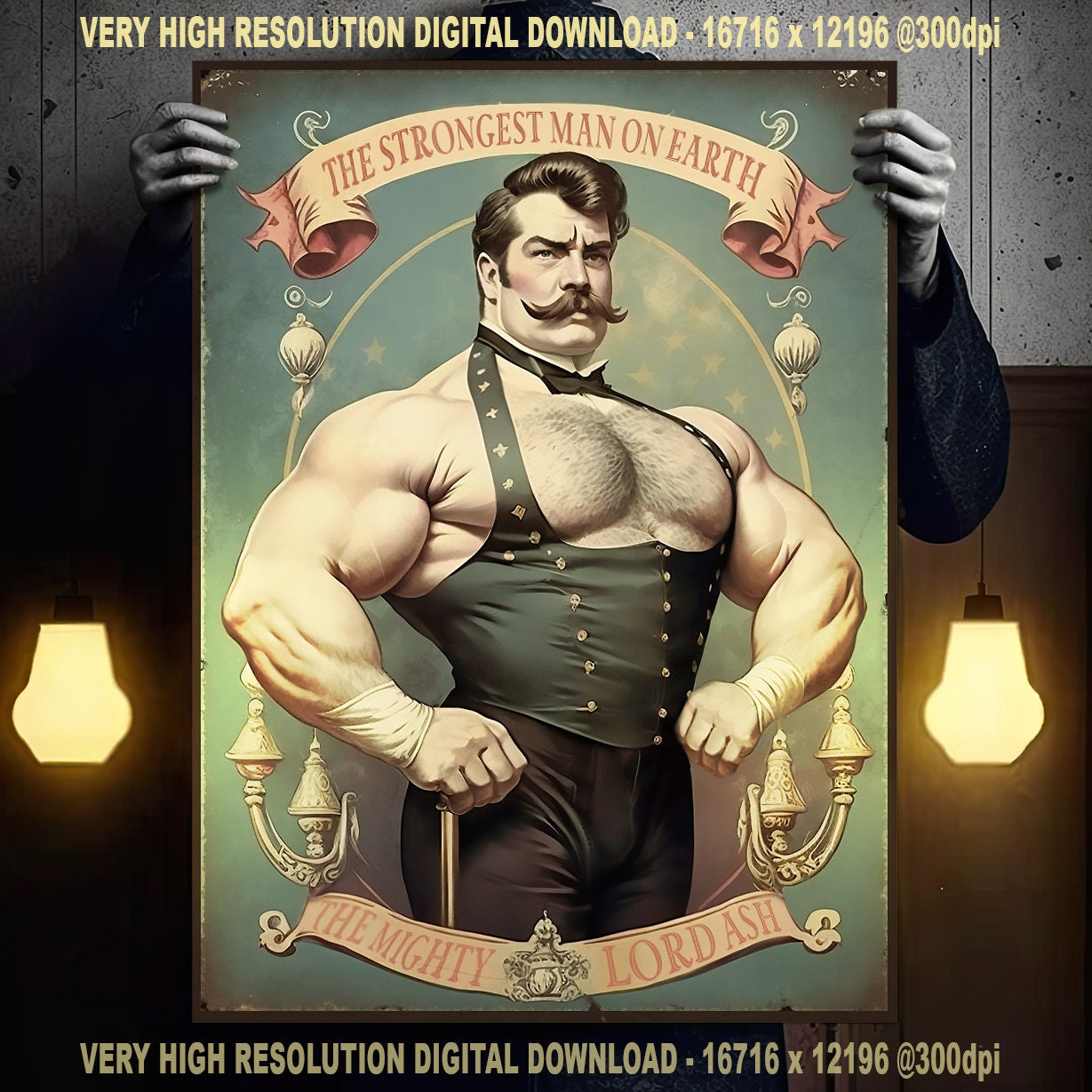In this picture, a person is holding a large poster with only their hands visible. The poster prominently features a highly detailed and muscular man with slicked-back, old-fashioned hairstyle and a long handlebar mustache. He is adorned in a sleeveless top and black pants, revealing a hairy chest, and accessorized with a bow tie. The man is framed against a teal background. At the top of the poster, a banner reads "The Strongest Man on Earth," and below the image is the caption "The Mighty Lord Ash." Both the top and bottom of the poster include text that states, "Very high-resolution digital download 16716 x 12196 at 300 DPI." The scene is complemented by lamps on either side of the person holding the poster, indicating a setting rich in detail and context.